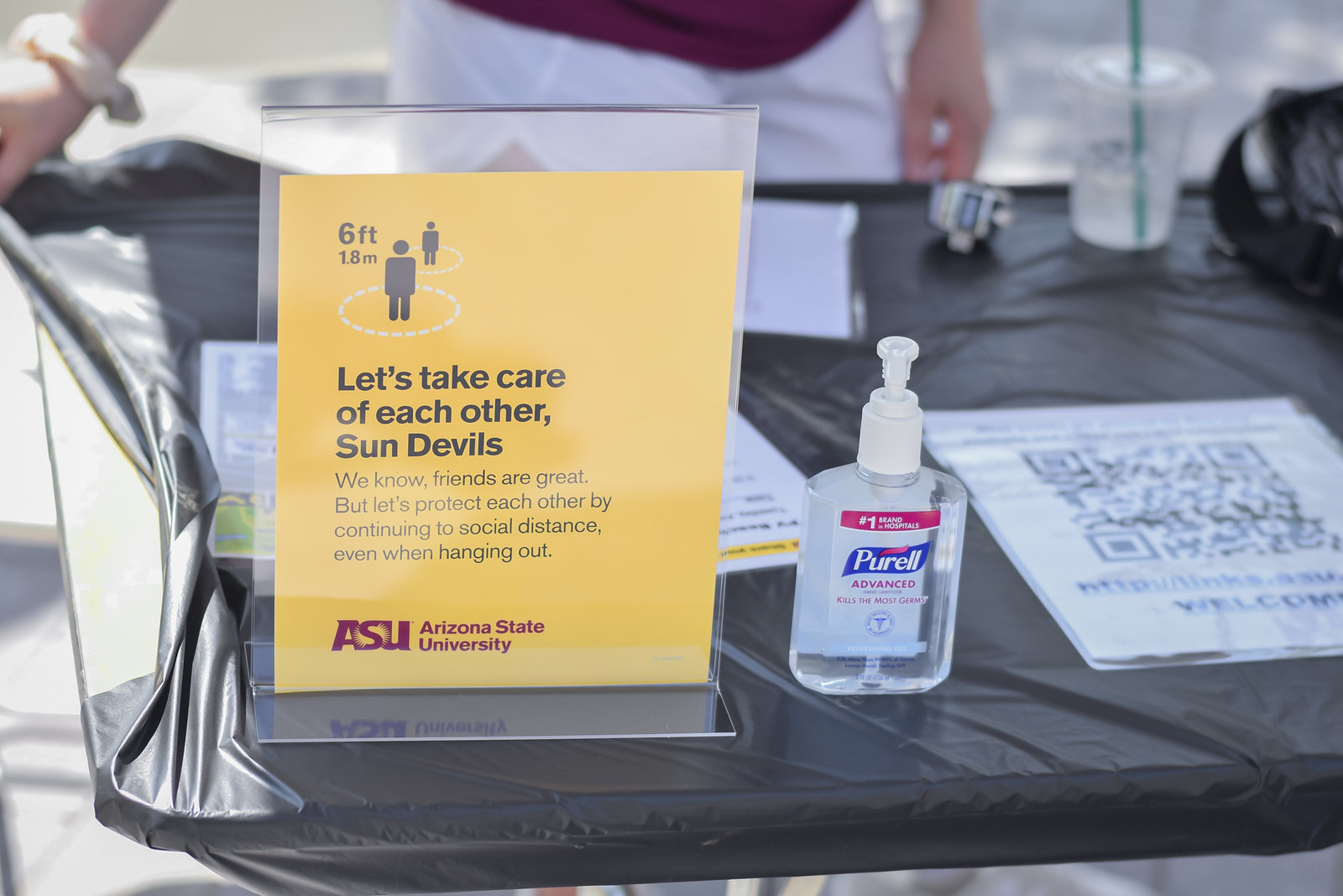This is a detailed close-up image of a black table, covered with a black tablecloth. In the background, somewhat blurry, a person is visible, identifiable only by the tops of their thighs in white pants and the bottom of a maroon-colored shirt. One of their hands rests on the corner of the table, while the other, possibly adorned with a lizard or some sort of animal wrapped around the wrist, hangs by their side.

On the table, in a glass stand, there's a prominent yellow sign that reads: "Let's take care of each other, Sun Devils. We know friends are great, but let’s protect each other by continuing to social distance even when we hang out." At the bottom of this sign, it mentions "Arizona State University" in red letters, indicating it's a social distancing notice related to COVID-19.

Next to the yellow sign, on the left stands a bottle of Purell hand sanitizer, reinforcing the health and safety measures. To the right of the sanitizer, a laminated sheet containing a large QR code is visible, intended for scanning, likely to learn more about the university's COVID-19 measures. In the background to the right, there is a water cup with a green straw and a counting device, presumably used to track the number of individuals present.

This setup seems to represent an information table for Arizona State University, primarily focused on social distancing and health precautions.